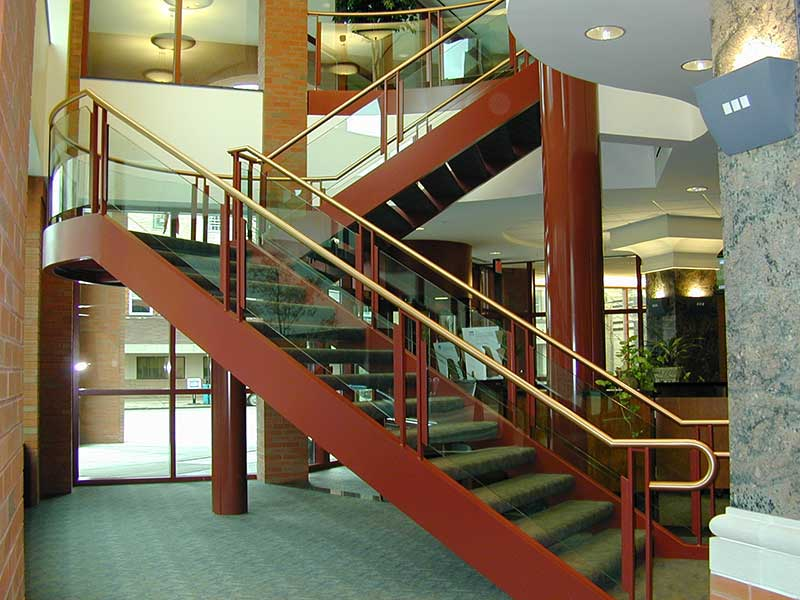The image showcases the interior of an upscale business building, featuring a prominent two-story staircase. The stairs, carpeted in a greenish-gray hue, begin with a single flight that ascends and turns at a small circular landing before continuing upwards. The staircase is intricately designed, with gold handrails and red metal railings that include glass panels for added safety. The steps themselves lack the vertical risers, creating an open, airy feel. The surrounding walls are primarily brick, with sections painted white or adorned with fake gray marble pillars housing wall sconces for illumination. The office features green carpet throughout, including on the staircase, and boasts a generous four-pane window at the front, which allows natural light to flood the space. A receptionist's desk laden with live plants is positioned prominently under the staircase and near the window, contributing to the welcoming atmosphere of the area.